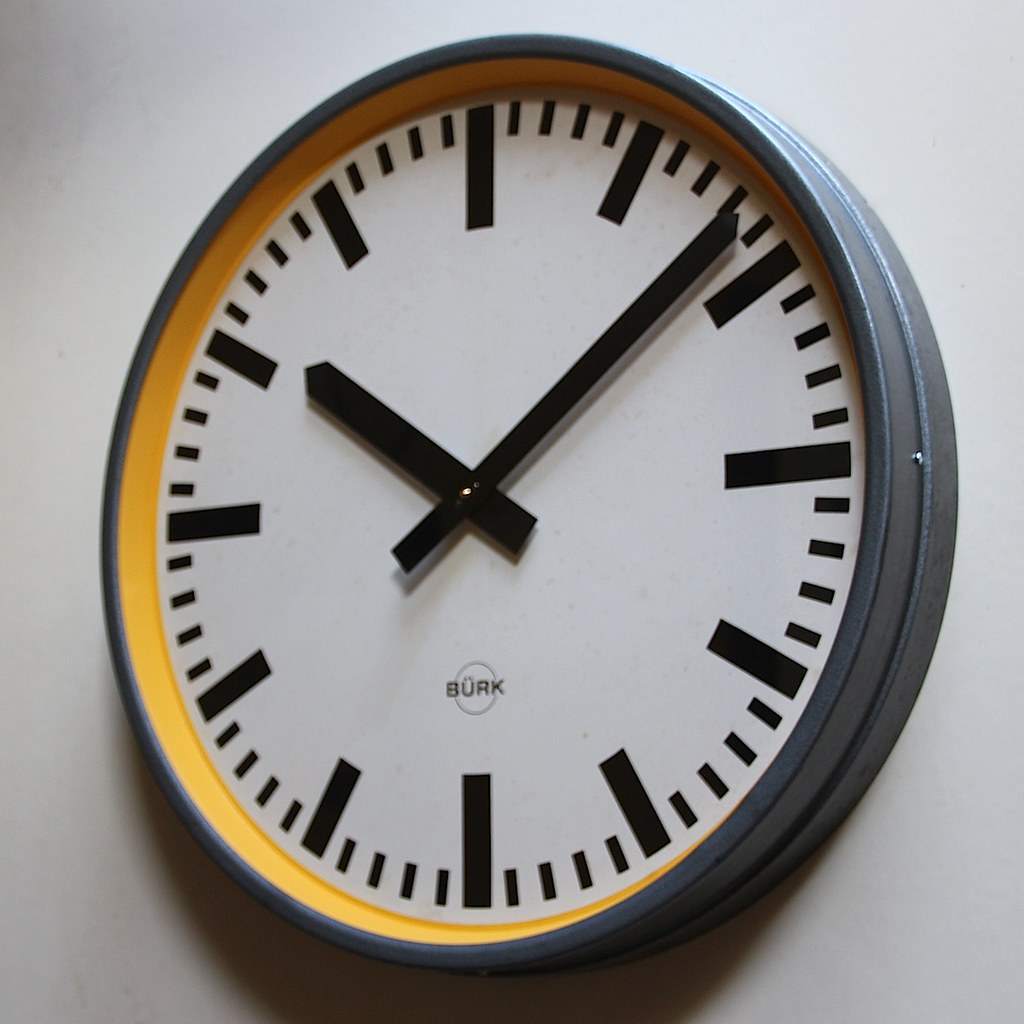The photographic image depicts a round, metallic clock with a nuanced blend of design elements mounted on a stark white wall. The clock’s outer casing is fashioned from a narrow, steel-like material, adorned with rivets along its side. This case frames an inner yellow rim that encircles the clock’s white face. The clock face features prominent black line ticks to mark the hours, with smaller lines in between to denote the minutes; no numeric values are present. Two black hands indicate the time, showing approximately 10:08, with a distinct absence of a seconds hand. Positioned near the bottom of the clock face is a tiny logo, "BURK," inscribed in light black letters within a small circle. The clock casts a subtle shadow downward, suggesting illumination from an overhead light source.